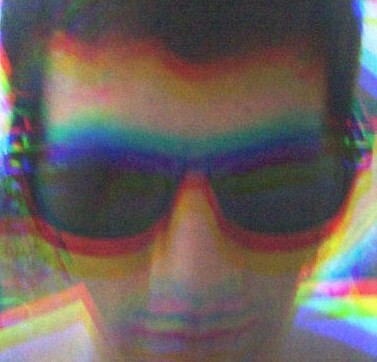The image depicts a close-up, slightly blurry photograph of a young male, who appears to be around 20 years old, with dark hair and wearing black sunglasses. His face occupies most of the frame, and he has a neutral expression. The man has no shirt on, as indicated by the visibility of his bare shoulders extending beyond the sides of his cheeks. A distinct rainbow, prism-like effect outlines the edges of his features, creating colorful halos throughout the image. The outlines include red below his hairline, blue and green above his sunglasses, and red underneath them, contributing to a surreal, almost psychedelic ambiance. This colorful aura extends beyond his figure, blending with background hues of purple, blue, white, and yellow, further emphasizing the image's blurred and dreamlike quality.